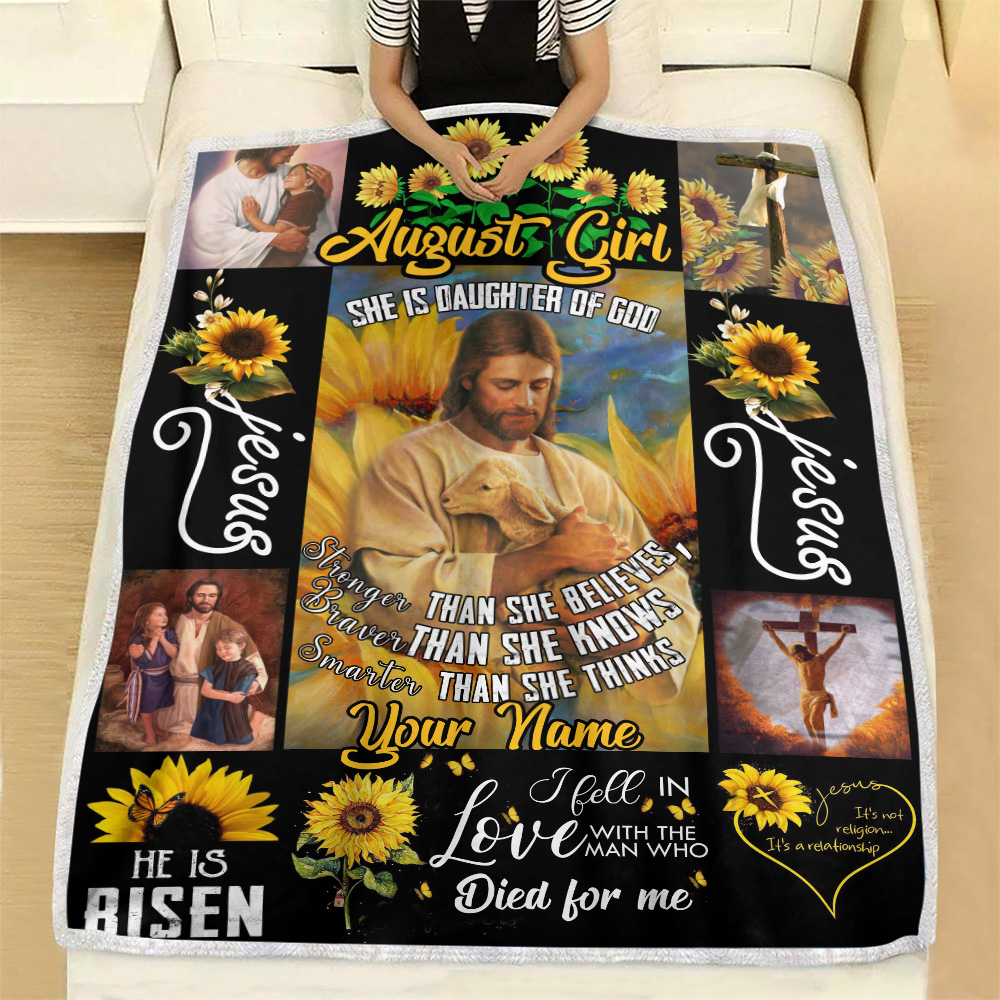In this indoor photograph, a woman is seen sitting upright in a white bed, her torso adorned with a black vest over a short-sleeve, horizontally-striped black and white shirt. The headboard of the bed is white, with its lower part visible in the image, and a light brown hardwood floor frames both sides of the bed. Positioned in the upper left corner is a white nightstand or dresser. 

The focal point of the image is a highly detailed and customized religious blanket that she is covered in. This blanket is vibrant with colors such as brown, white, tan, green, orange, yellow, black, gray, and blue, and is adorned with a multitude of images and text. The centerpiece of the blanket features a large rectangular depiction of Jesus holding a lamb, with the words "August girl, she is the daughter of God, stronger, braver, smarter than she believes, than she knows, than she thinks, your name" arranged around Him. This text suggests that the blanket can be personalized with different names and possibly different months.

Various other images of Jesus adorn the blanket: in the upper left corner, Jesus is seen with a child; in the upper right corner, He is caressing a girl; and in the bottom left corner, He is holding two children. The blanket also features images of sunflowers, a cross draped with a robe, and Jesus on the cross. Additional phrases and decorations include "He is risen" with a daisy and butterfly in the bottom left, and a heart with a daisy stating "Jesus, it's not religion, it's a relationship" in the bottom right. The blanket is bordered by multiple squares and rectangles, each containing different religious images, including the word "Jesus" flanked by daisies on either side in the middle of the blanket, reinforcing its personalized and religious theme. 

The overall impression is that the photograph serves as an advertisement for a customizable, religious-themed blanket, richly decorated with symbolic iconography and uplifting messages.